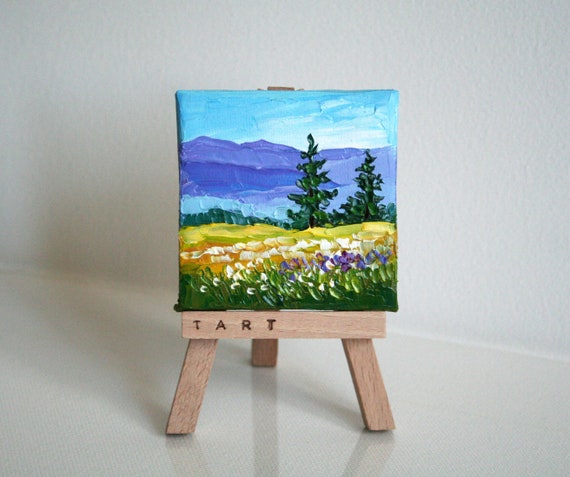The image features a small, light tan wooden tabletop easel with slightly splayed legs, set against a gray background. The easel has the word "TART" engraved in black on the horizontal support bar. On the easel rests a colorful, unframed watercolor painting. The painting depicts a vibrant landscape scene: blooming wildflowers of various colors, green grass in the foreground, and purple-hued mountains with peaks and valleys in the background. To the right, two tall evergreen pine trees stand before a serene blue lake. Above, a sky with blue and white clouds adds depth to the scene. The photograph captures the entire setup in a realistic, detailed manner typical of product photography.